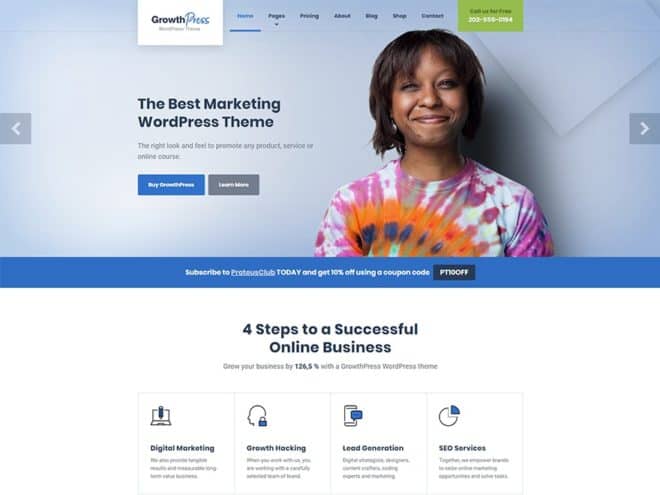The image features a web interface labeled "GripPress" prominently at the top, enclosed within a white box. To its right, there's a menu with seven clickable options, though the text is too blurry to decipher. Adjacent to the menu, a green box is visible, likely containing a phone number, although the details are unclear. Below the header, the tagline reads, "The best marketing WordPress theme," followed by a description highlighting its suitability for any product, service, or course. Two buttons are positioned beneath this text—one blue and one gray.

On the right side of the image, there is a portrait of a Black woman with chin-length hair, wearing a vibrant purple, orange, and white tie-dye shirt. Below her picture, a blue box invites users to "Subscribe to something club today and get 10% off using the coupon code," promoting a special offer. Further down, the image is divided into four sections titled "Four steps to a successful online business," with brief descriptions under each section: "Digital marketing," "Growth tracking," and "Lead generation."